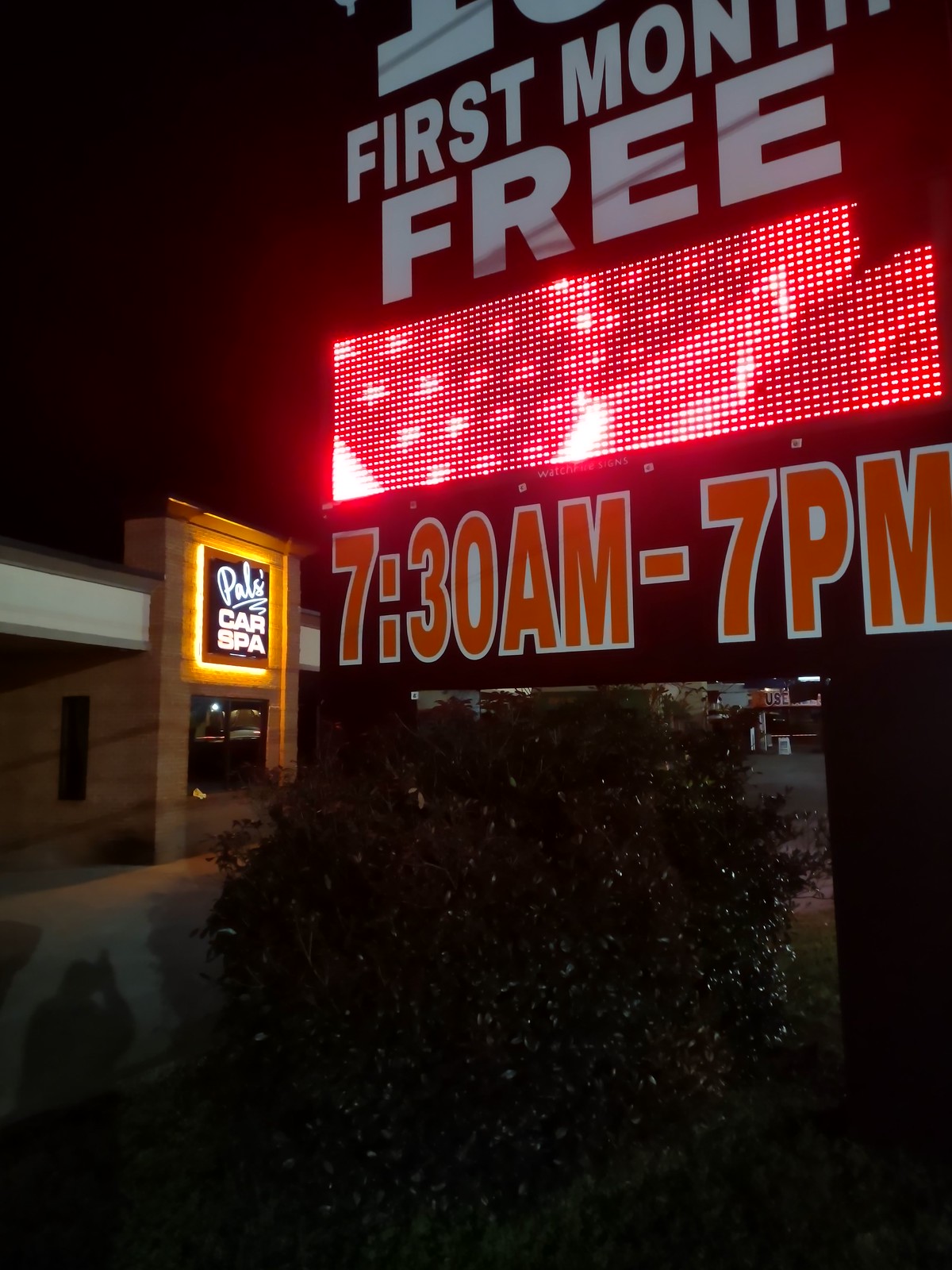This nighttime color photograph captures a fragmented view of a commercial sign. The top of the sign is cut off, yet clearly displays the bold, all-caps inscription "FIRST MONTH FREE" in striking white letters. Below this text, a vivid red LCD screen prominently features an image of an American flag. Further down, the operational hours "7:30 A.M. to 7 P.M." are visible in contrasting white text. A dense, leafy bush occupies the space directly beneath the signage. To the left, another sign reads "Powell's Car Spa," distinctively black with a yellow neon outline. The scene is devoid of people, animals, vehicles, water, and airplanes, presenting a quiet urban nightscape.